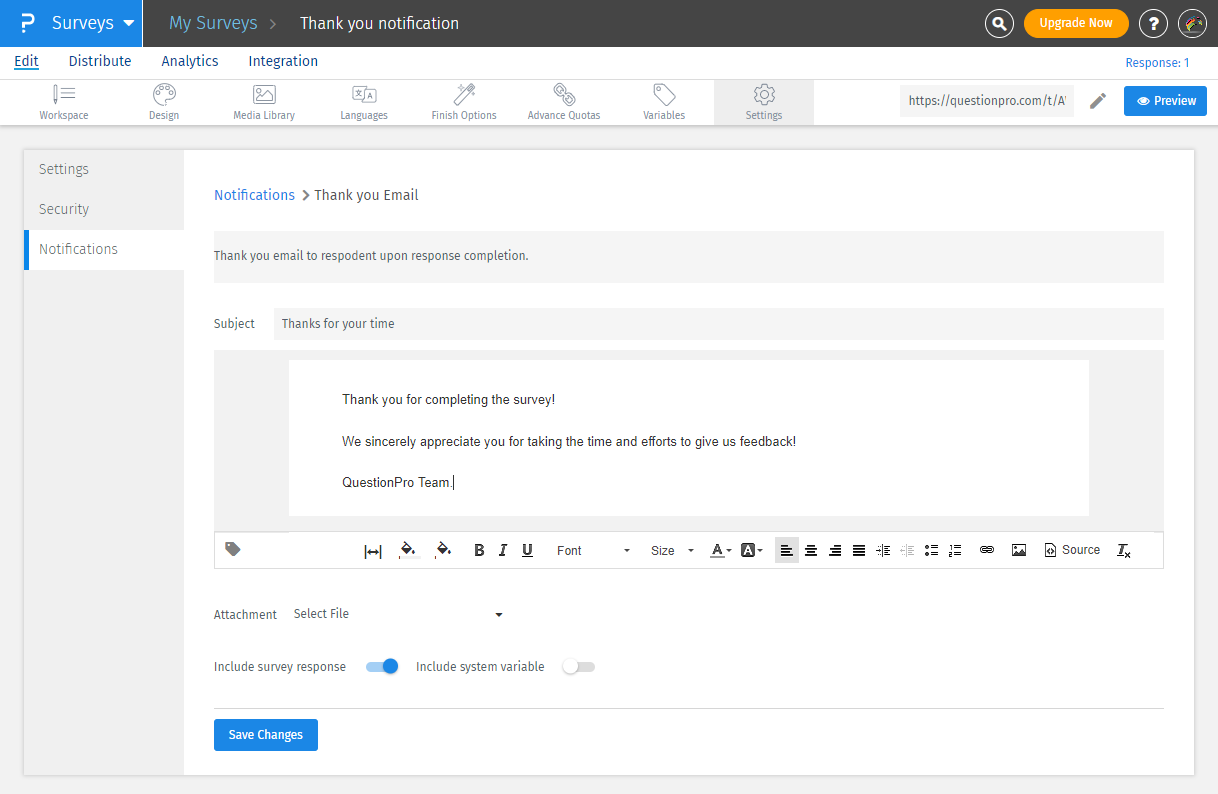This image showcases the interface of a survey management tool on a website, primarily displaying a detailed view of a "Thank You" notification setup. The interface background features a clean palette of white and gray shades.

In the top left corner, a prominent blue box with a white question mark and the word "Surveys" stands out. Across the top of the screen runs a sleek black bar that includes several interactive elements. "My Surveys" is highlighted in blue, next to a "Thank You Notification" label. Additionally, the bar features a magnifying glass icon for search functionality and an "Upgrade Now" button in a noticeable orange oval shape, accompanied by another question mark icon.

Below this, a range of navigational and functional options are presented in blue text, including "Edit," "Distribute," "Analytics," and "Integration," with "Edit" being underlined to indicate the current selection. Adjacent to "Response," a counter displays the number "1."

On the left side, within a gray shaded sidebar, detailed categories are listed: Workspace, Design, Media Library, Languages, Finish Options, Advanced Quotas, Variables, and Settings. The Settings category is highlighted, revealing subcategories of Security and Notifications, with Notifications currently selected.

The main section of the interface elaborates on the "Thank You" email configuration. It mentions an email notification that is sent to respondents upon survey completion. The subject line reads "Thanks for your time," and the email content expresses gratitude: "Thank you for completing the survey. We sincerely appreciate you for taking the time and efforts to give us feedback! - QuestionPro Team." There is also an option to attach a file, labeled "Select File," and an option to include the survey response, which is turned on. At the bottom, a "Save Changes" button is highlighted in blue, ready for user interaction.